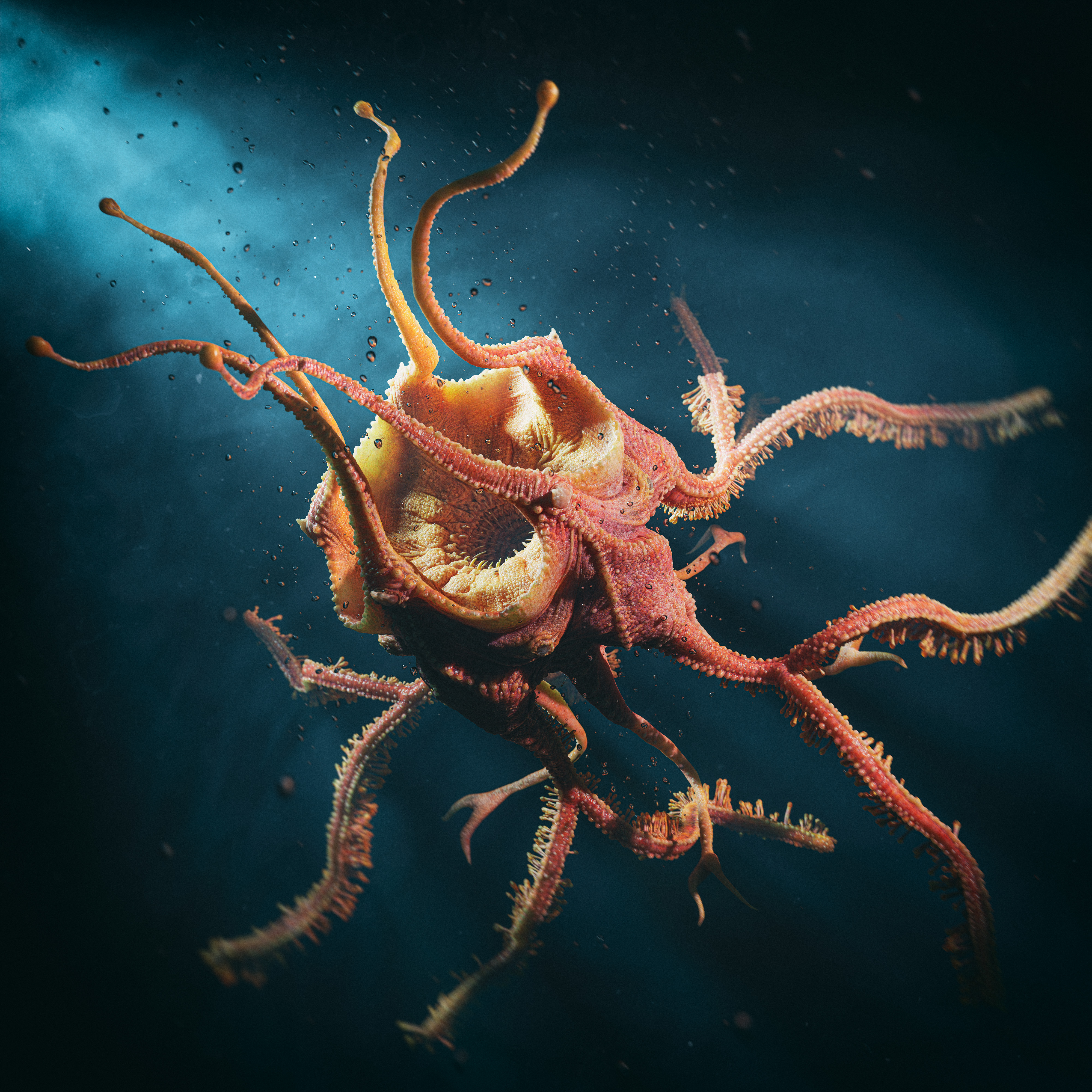This vibrant underwater photograph showcases an octopus deep in the sea, highlighted against a dark, deep blue background with rays of light streaming in from the top left corner, illuminating the scene. The octopus, with its striking orangey-red tentacles adorned with a light yellowish fringe, is fully outstretched, revealing its magnificent form. Tiny air bubbles surround the creature, suggesting movement as it explores or breathes. The intricate details of its anatomy are visible, including tentacles with variations of red and yellow, ending in forked or rounded tips. Some tentacles have spiky protrusions, adding a textured look to its elegant display. In the center of its body, there is a lighter yellow swirling pattern, and a large, open mouth, resembling a deep hole, adds to its mysterious allure. The scene captures the solitary magnificence of the octopus, beautifully set against a backdrop of dark and light blue hues, with no other objects in sight.